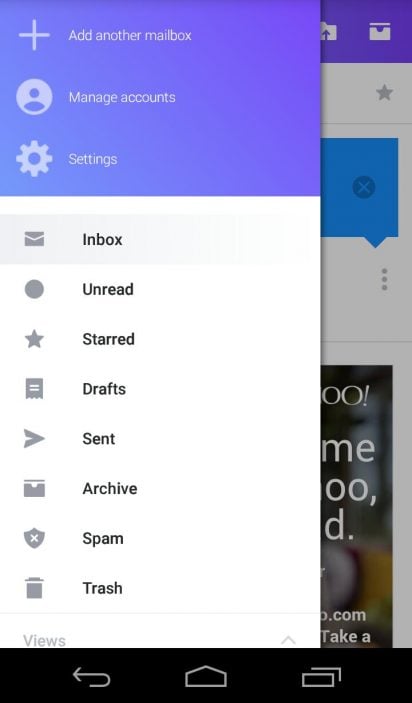The image depicts a screenshot of a digital interface, likely from a smartphone or tablet, displaying a menu from the Yahoo Mail application or mobile website. At the top of the menu, three options are highlighted in purple:

1. A plus symbol with the text "Add another mailbox".
2. An icon depicting a user with the text "Manage accounts".
3. A gear symbol labeled "Settings".

Directly below these options, a series of mail management options are listed, each accompanied by a distinctive icon:

- "Inbox" with a red mail symbol.
- "Starred" with a star symbol.
- "Drafts" without an additional icon.
- "Sent" with an arrow symbol.
- "Archive" with a folder symbol.
- "Spam" with a shield symbol marked with an X.
- "Trash" with a trash can symbol.

At the bottom of the screen, a black navigation bar displays three icons:
- A back arrow for returning to the previous screen.
- A home button for returning to the home screen.
- A square indicating the option to view multiple windows or apps.

In the background behind the menu, a partially obscured page is visible. Although the details of this background page are unclear, it contains some text and an image, suggesting that the user was previously viewing this content. The overall design and recognizable icons suggest that this is a Yahoo Mail interface, specifically showing the mail settings pane.